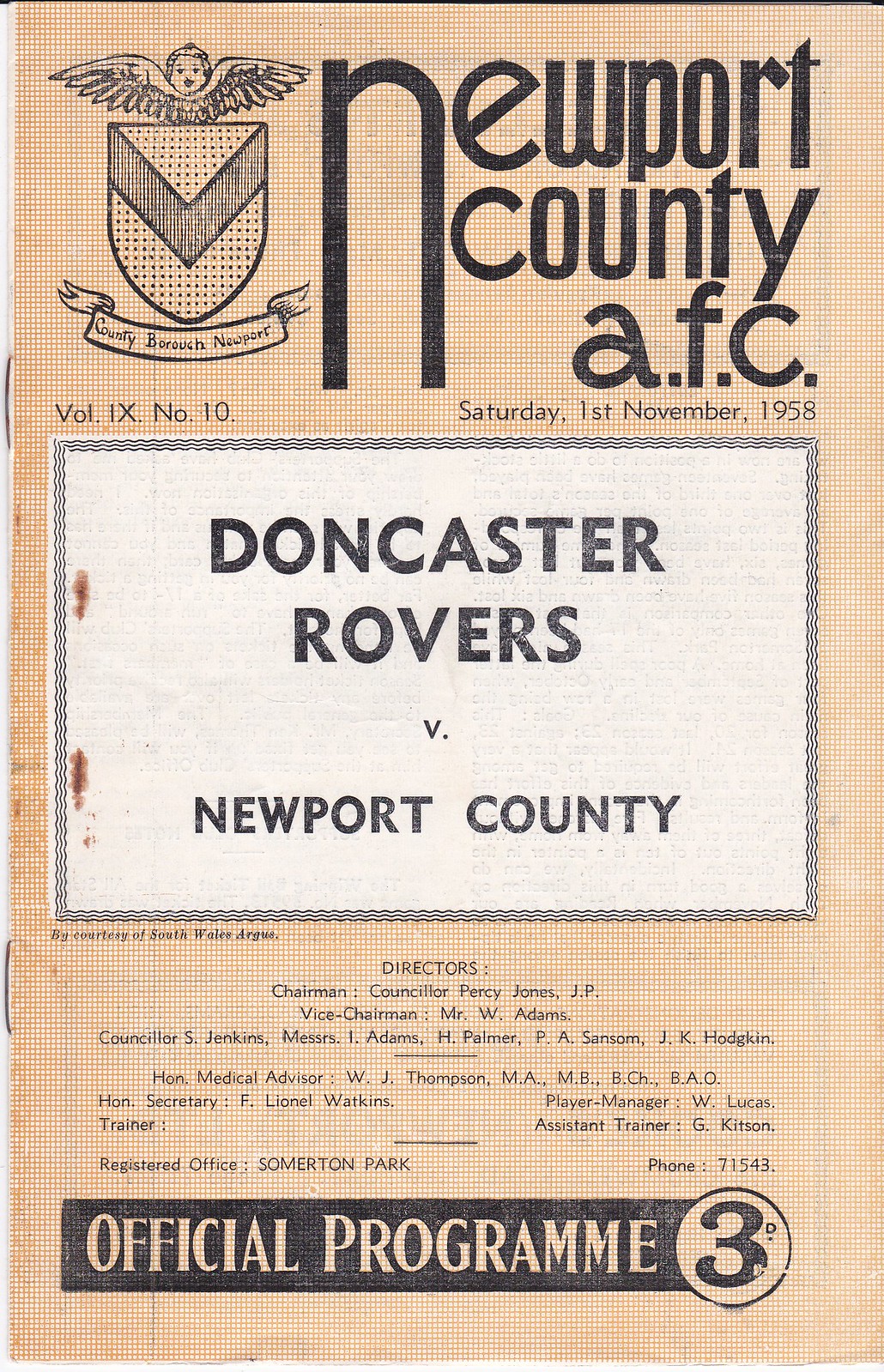The image is a rectangular program brochure, measuring approximately 6 inches tall and 3 to 4 inches wide. The background has a pale pink or peachy tone with a texture reminiscent of straw.

At the top left of the brochure, there is a detailed emblem consisting of a shield with wings at the top, a human face, and a cherub above it. Below the shield, a banner reads "County Borough Newport." Below the emblem are the details "V-O-L. I-X N-O. 10" in small black font. To the right of the emblem, in bold black print, there's the text "Newport County A.F.C.," with the particularly large 'N' spanning three rows. Directly below, the date "Saturday, 1st November 1958" is written in the same small black font as the volume and issue number.

In the center of the brochure, there is a white rectangle with a black outline. Inside this rectangle, the text reads "Doncaster Rovers vs. Newport County" in bold black print. Below this, there are lists of team officials including the Chairman Percy Jones, J.P., Vice-Chairman W. Adams, and other counselors and officials like I. Adams and P.A. Sampson. There is also mention of roles such as the Player Manager W. Lucas, Assistant Trainer G. Kitson, and the Registered Office at Somerton Park, with a contact phone number 71543.

At the very bottom of the brochure, a black rectangular box contains the text "Official Program" in pale pink lettering, consistent with the rest of the brochure's background color. Next to this text, there is a black number 3 inside a circle.

Overall, the brochure provides detailed information about a sporting event held on November 1, 1958, between Doncaster Rovers and Newport County, emphasizing club details and official roles.